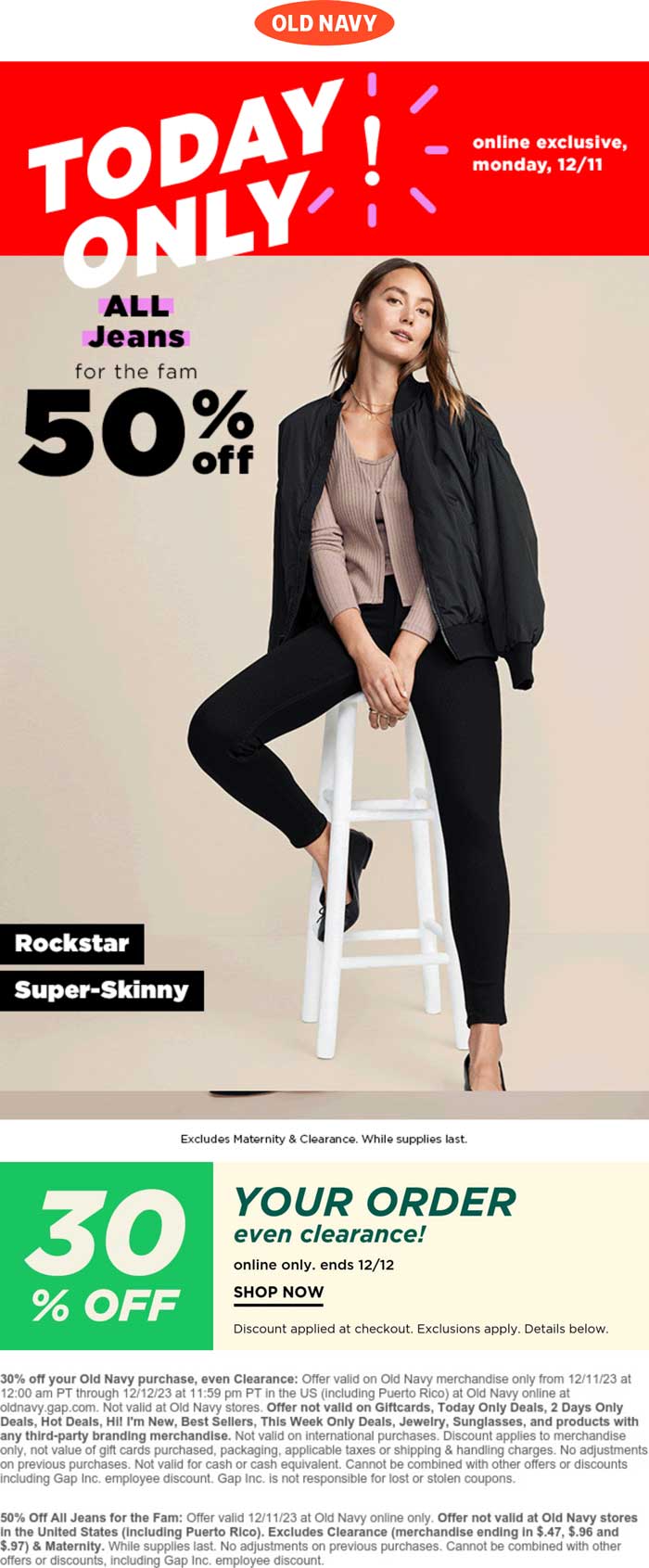This image features a desktop screenshot of an Old Navy advertisement. The top of the ad prominently displays a "Today Only" message on a vibrant red background, emphasizing the urgency of the offer. It highlights an "Online Exclusive for Monday 12-11."

Below the promotional text, the ad showcases a photo of a stylishly dressed woman. She is seated on a tall white stool, exuding a confident demeanor. The woman, who has auburn brown hair and a slightly tanned, Caucasian complexion, is attired in a sophisticated black blazer over a light brown blouse. Her ensemble is complemented by form-fitting black pants, identified as the Old Navy "Rockstar Super Skinny" jeans, and black flat shoes.

Further down, the ad announces, "All jeans for the fam, 50% off," suggesting a family-wide discount on denim. It also includes a note clarifying that the discount excludes maternity and clearance items, and is available while supplies last.

At the bottom of the ad, a green square highlights another offer: "30% off your order, even clearance," valid online only until 12-12. There's also a prompt urging customers to "Shop Now," with a reminder that the discount will be applied at checkout and that exclusions apply, with details provided below.